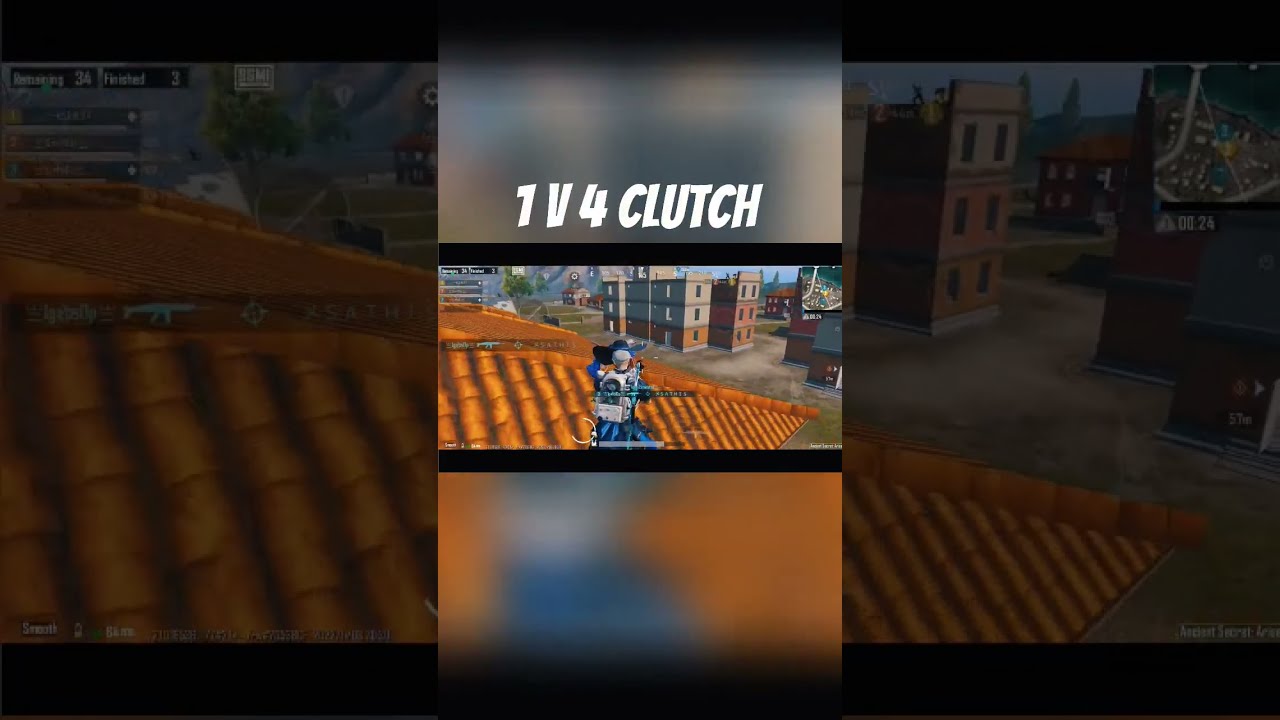The image is a detailed screenshot of a video game with cartoonish graphics, featuring a central character who appears to have a gun and is depicted in a futuristic style. The character, who has a white backpack and armor, stands on a terracotta rooftop, likely in the middle of a 1 vs. 4 clutch scenario as indicated by the white label at the top of the image. The background reveals a cityscape with multiple buildings, including what seem to be traditional apartment-style structures and office high-rises, along with some trees. The central screenshot is set within a larger, blurred rendition of the same scene, bordered in shades of green and gold. Icons such as a map and an ammo indicator are visible on the screen. The player character wears a blue outfit, including a blue hat with a white brim, and looks into the distance amidst the diverse urban backdrop.